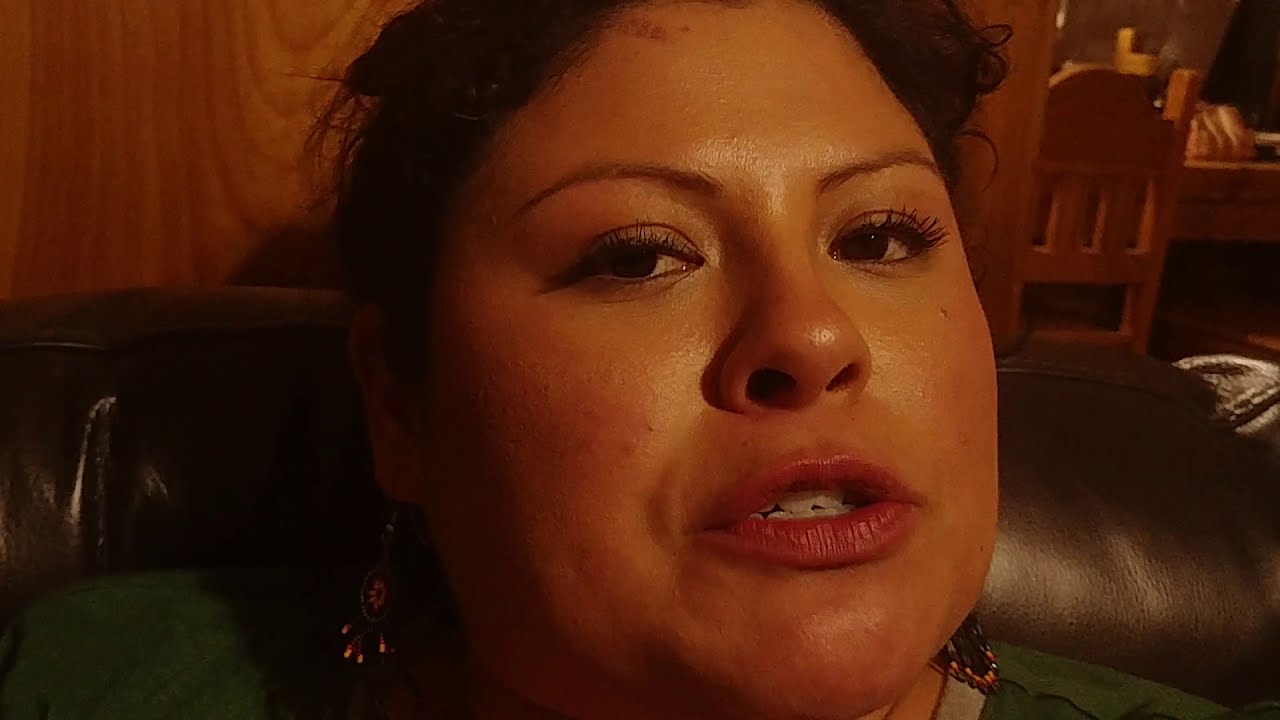The photograph is a close-up, landscape-oriented image of a Latina woman with olive-toned skin and dark, backlit hair that's pulled behind her shoulders. She is wearing earrings that are oval with dangling elements and a green shirt with a gray border around the neckline. The woman's mouth is partially open, her teeth together as if caught mid-sentence. She has dark eyes, shaped eyebrows, long eyelashes, mascara, and light red lipstick. She is seated on a dark brown leather couch. In the background, a brown wooden wall is visible on the left, and on the right, there is an open doorway revealing a wooden chair pushed against a wooden table with indeterminate items on it. Her expression and posture suggest she is engaging directly with the viewer.